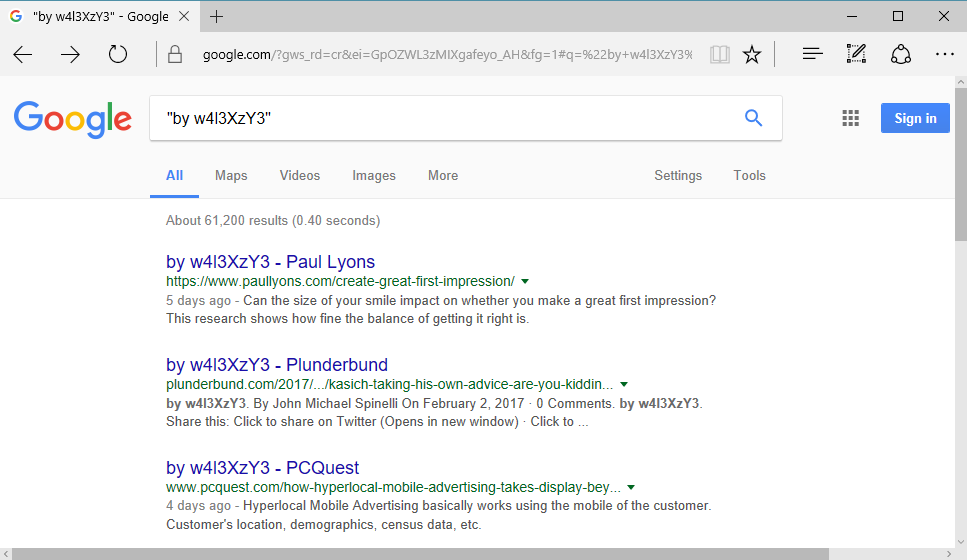Caption: 

The image captures a Google search results page featuring the query "by w4i3xzy3." At the top, the recognizable Google logo sits adjacent to the search bar, which contains the search term. Below the search bar are various tabs labeled 'All,' 'Maps,' 'Videos,' 'Images,' 'News,' and 'More,' with 'All' being selected. The page indicates approximately 61,000 results found within 0.4 seconds. 

The first search result displays a link to a page titled "w4i3xzy3 Paul Lyons" with the URL "paullyons.com", paired with a snippet from 5 days ago, questioning if the size of one's smile could impact making a great first impression, suggesting the delicate balance involved in achieving this. The second result features the title "blunderbund," linking to "blunderbund.com," and includes a snippet about Kasik taking his own advice dated February 2nd, 2017, with no comments, and a prompt to share on Twitter in a new window. The third result is titled "by w4i3xzy3 PCquest" with a URL linking to "PCquest," discussing how hyper-local mobile advertising utilizes customer's mobile data, including location, demographics, and census information. 

On the right side, a blue 'Sign in' button can be seen. The page background is white, with black text and hyperlinked text highlighted in blue and green. The overall design of the search result interface remains clean and straightforward, consistent with Google's typical layout.